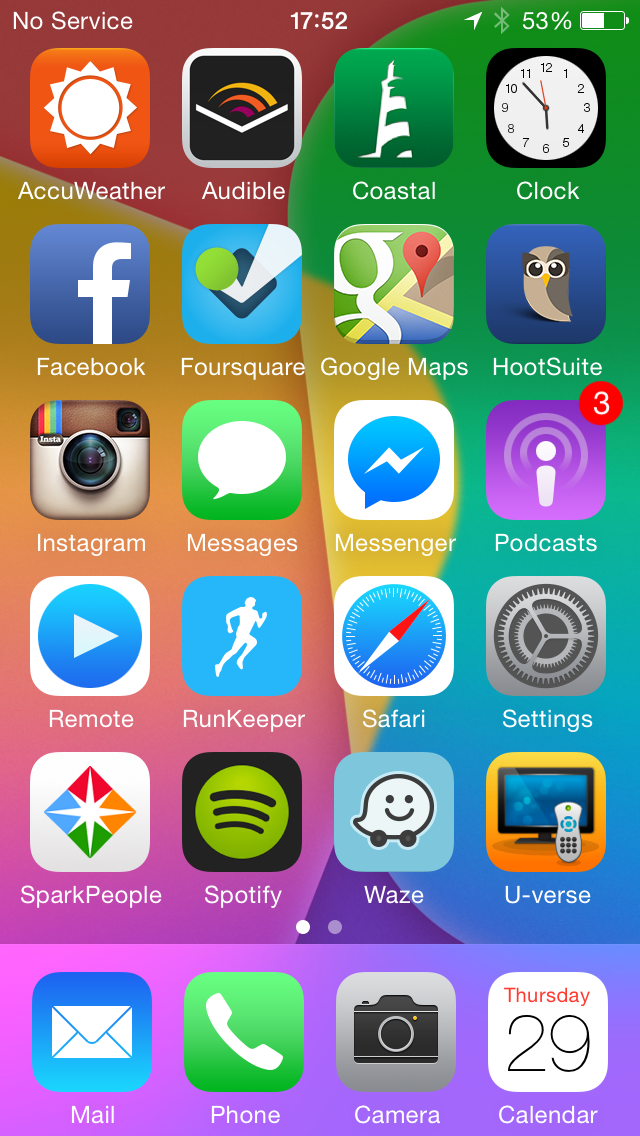The image showcases a long, rectangular screen featuring a gradient background transitioning through a spectrum of colors, from pale blue and purple to dark khaki and murky red, with hints of green interspersed. This vibrant display serves as the backdrop for a collection of app icons, arranged in a grid format, likely from a smartphone or computer. Each icon is accompanied by its respective app name, with familiar ones such as Facebook, Google Maps, Messenger, Messages, Instagram, Spotify, Phone, Mail, and Camera standing out. In the bottom right-hand corner, the current date is prominently displayed, while the upper right-hand corner features a clear and easily readable clock. The center of the top edge also indicates the current time in text, and an indication of "No Service" is visible, humorously reminiscent of broadband connection issues.